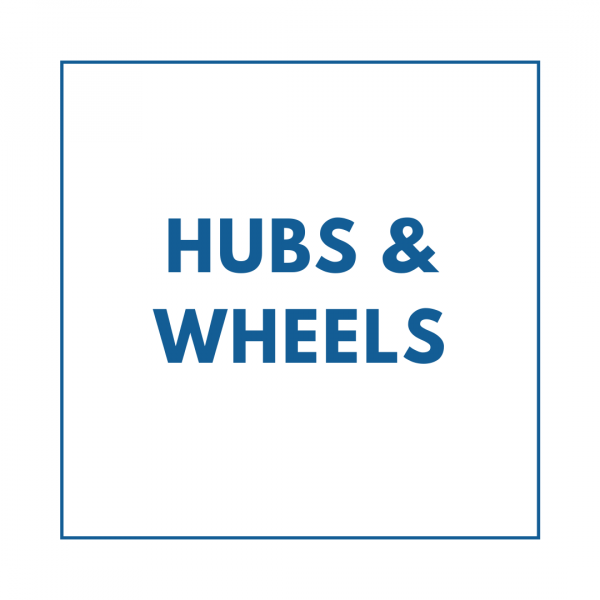The image is a simple PNG text file featuring a minimalist design. It displays a vertical, thin blue border forming a rectangle approximately 4 inches wide by 5 inches tall against a white background. Centered within this rectangle are two words: "HUBS" and "WHEELS," both written in large, all-capital, block-style font. The text is in a middle-tone, somewhat grayish blue. The word "HUBS" appears on the top line, followed by an ampersand, and below it, slightly larger, is the word "WHEELS." There are no other decorations, shadows, or embellishments within the image, creating a clean and straightforward look.